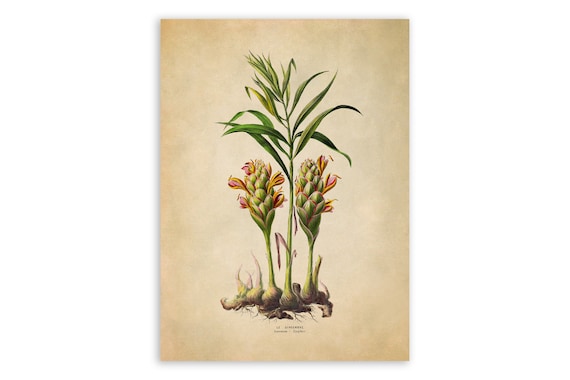This is an early 20th-century, naturalist-style drawing with a light beige, slightly faded background. It depicts six bulbs emerging from the brown soil. The bulbs are a whitish, light green color, with detailed roots extending downward. From the left, the first three bulbs have whitish-pink sprouts, gradually increasing in size. The fourth bulb transitions to a taller green stem with numerous green leaves sprouting out. The fifth and sixth bulbs display more pronounced growth, resembling corn stalks. These two plants feature reddish-orange flowers budding along their stems. The overall composition of the drawing is detailed and intricate, with the taller central plant boasting several narrow leaves and the shorter ones budding and blooming. The delicate and herbal nature of this artwork, combined with the faded paper, suggests it's a meticulously documented botanical illustration, with tiny, illegible lettering likely indicating the genus or species of the depicted plant.